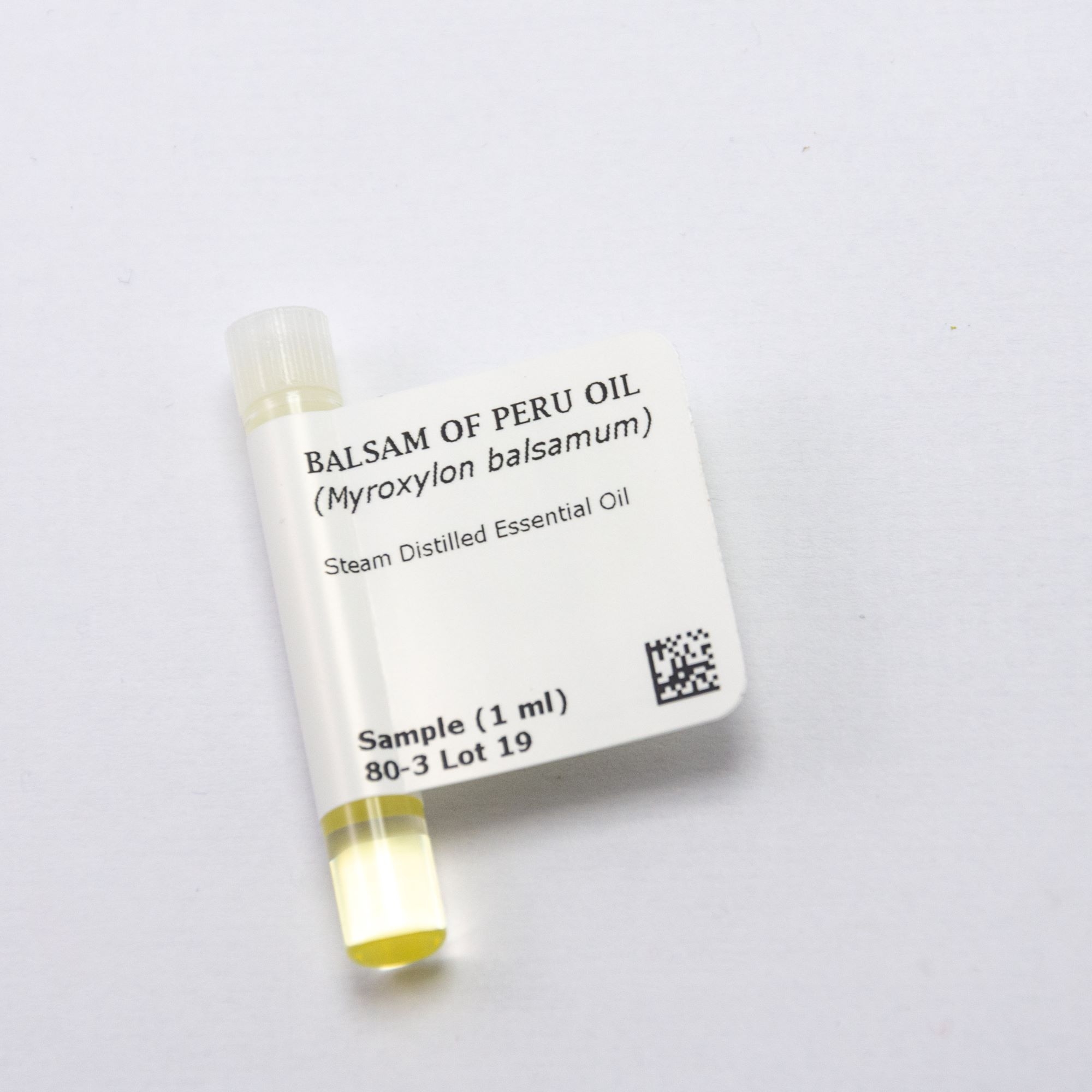This close-up product photograph showcases a very small, clear bottle with a ridged plastic cap, containing a light yellow liquid. The bottle is isolated against a white surface, potentially a table, suggesting a catalog or online shop listing. Wrapped around the main body, a white label prominently features black text. At the top, it reads "Balsam of Peru Oil," followed by "Myroxylon Balsamum," and "Steam Distilled Essential Oil." The label indicates that the bottle is a sample with a capacity of only 1ml, emphasizing its miniature size. Additional details on the label include the code "80-3 Lot 19" and a QR code in the bottom right corner, used for further identification of this specific sample.